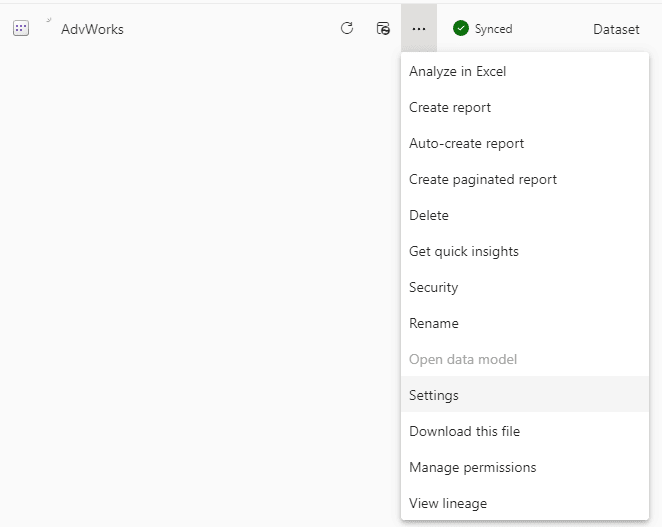This screenshot features a user interface with a grey background. In the top left corner, there's a square icon containing five miniature dark squares arranged with three on the top row and two on the bottom. To the right of this icon, the word "ADVWORKS" is displayed, with both the 'A' and 'W' capitalized. 

Continuing to the right, there are several icons and symbols: a refresh symbol, a folder symbol with a circle and a line through it, and a three-dot (ellipsis) symbol. The ellipsis symbol has been highlighted, opening a sub-menu with a white background that contrasts the grey of the main interface.

The sub-menu lists the following options from top to bottom:
1. Analyze in Excel
2. Create Report
3. Auto-Create Report
4. Create Paginated Report (or Paginated Report)
5. Delete
6. Get Quick Thought
7. Get Quick Insights
8. Security
9. Rename
10. Open Data Model (this option is not clickable and is shaded in grey)
11. Settings (highlighted with a grey box, indicating it is currently selected)
12. Download This File
13. Manage Permissions
14. View Lineage

Right next to the three-dot icon at the top, there is a green circle with a white checkmark inside and the word "Synced" spelled out next to it. Lastly, at the very top right corner, the word "Dataset" is displayed.